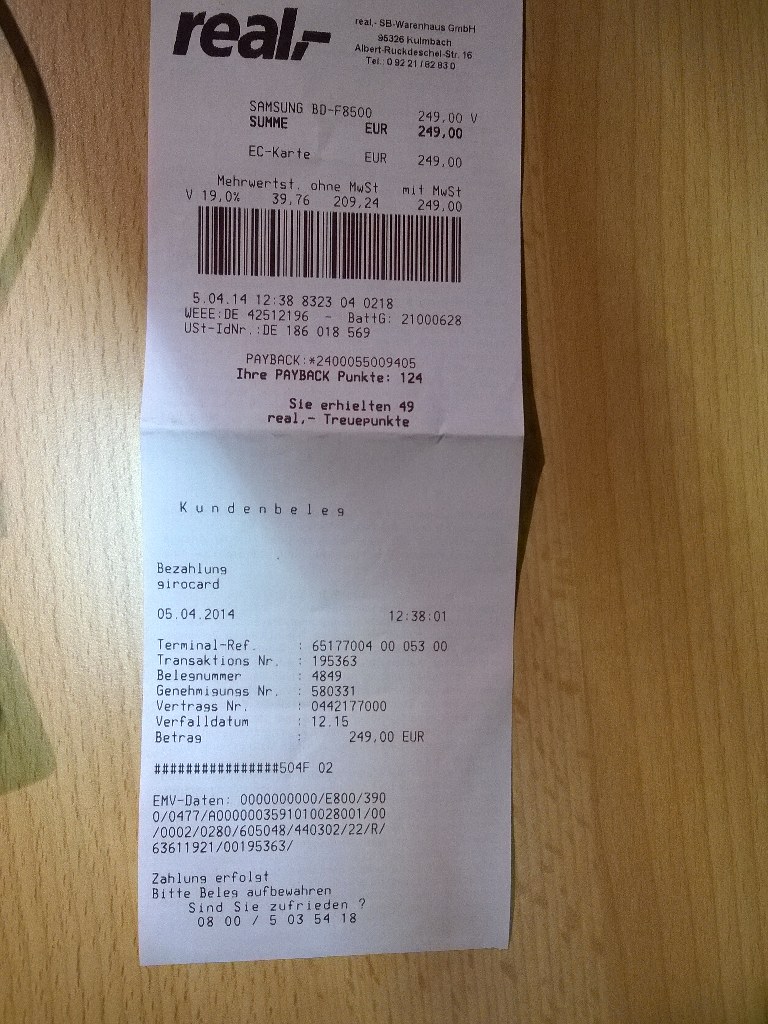This photograph captures a receipt printed on white paper with black ink, resting on a light blonde wood table. The image displays a distinct play of shadows and sunlight, with half of the receipt draped in shadow while sunlight illuminates the other half. The receipt is from a store named RealR, its name prominently displayed in bold black letters at the top. The document details the purchase of a Samsung electronic device, priced at $249. Additional nuances include text that appears to be in German and a shadow cast by another item, which is partially visible at the left edge of the frame.